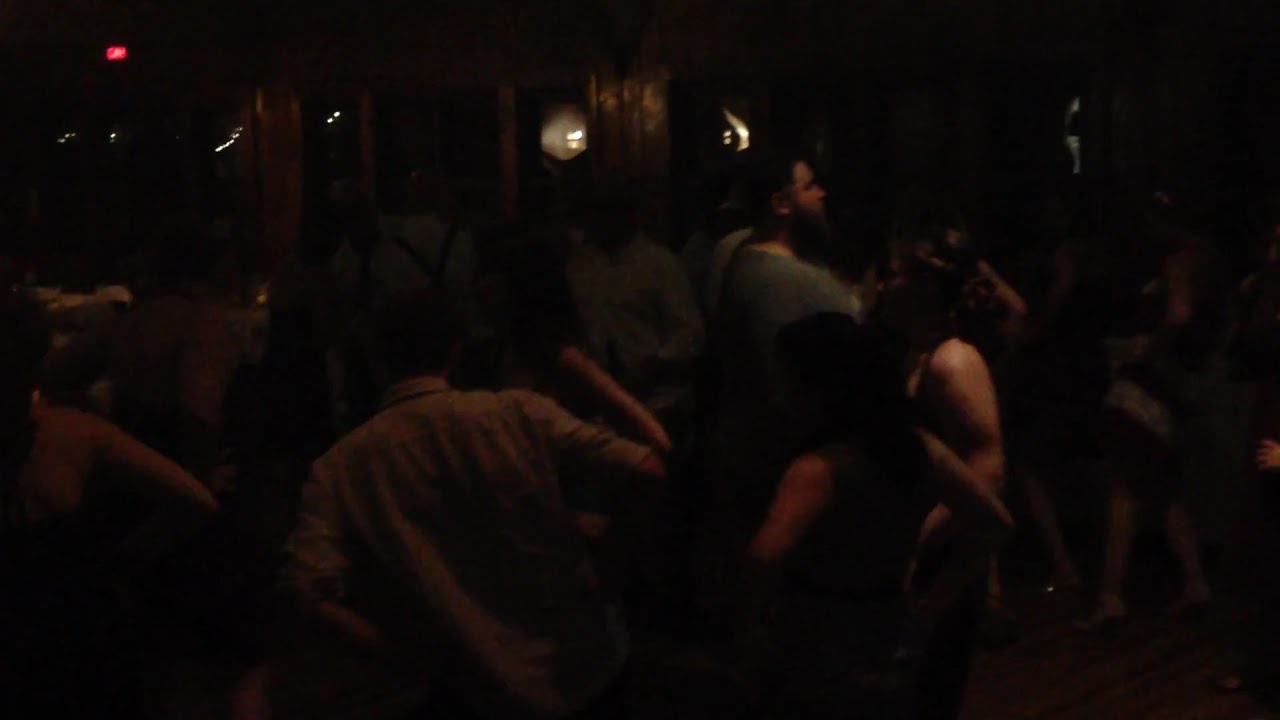In this dimly lit scene, likely set in a club or dancehall, young adults are gathered, engaging in lively dancing and socializing. The setting features a predominantly dark background with hints of brown walls and windows showing pitch-black darkness outside. Several people are discernible in the foreground: a man tilting his body to the left with his right arm raised, seemingly caught mid-dance move, and nearby, women with exposed shoulders, probably wearing tank tops or strapless dresses, their arms reflecting the sparse light. Another man in a gray t-shirt stands out among people, some of whom appear to be making energetic gestures like fist-pumping to the beat of the music. On the upper left side, a red illuminated exit sign glows, further emphasizing the low-light ambiance of the social event. Notably, the overall scene exudes a lively atmosphere reminiscent of a renaissance painting brought to life with modern-day revelers.